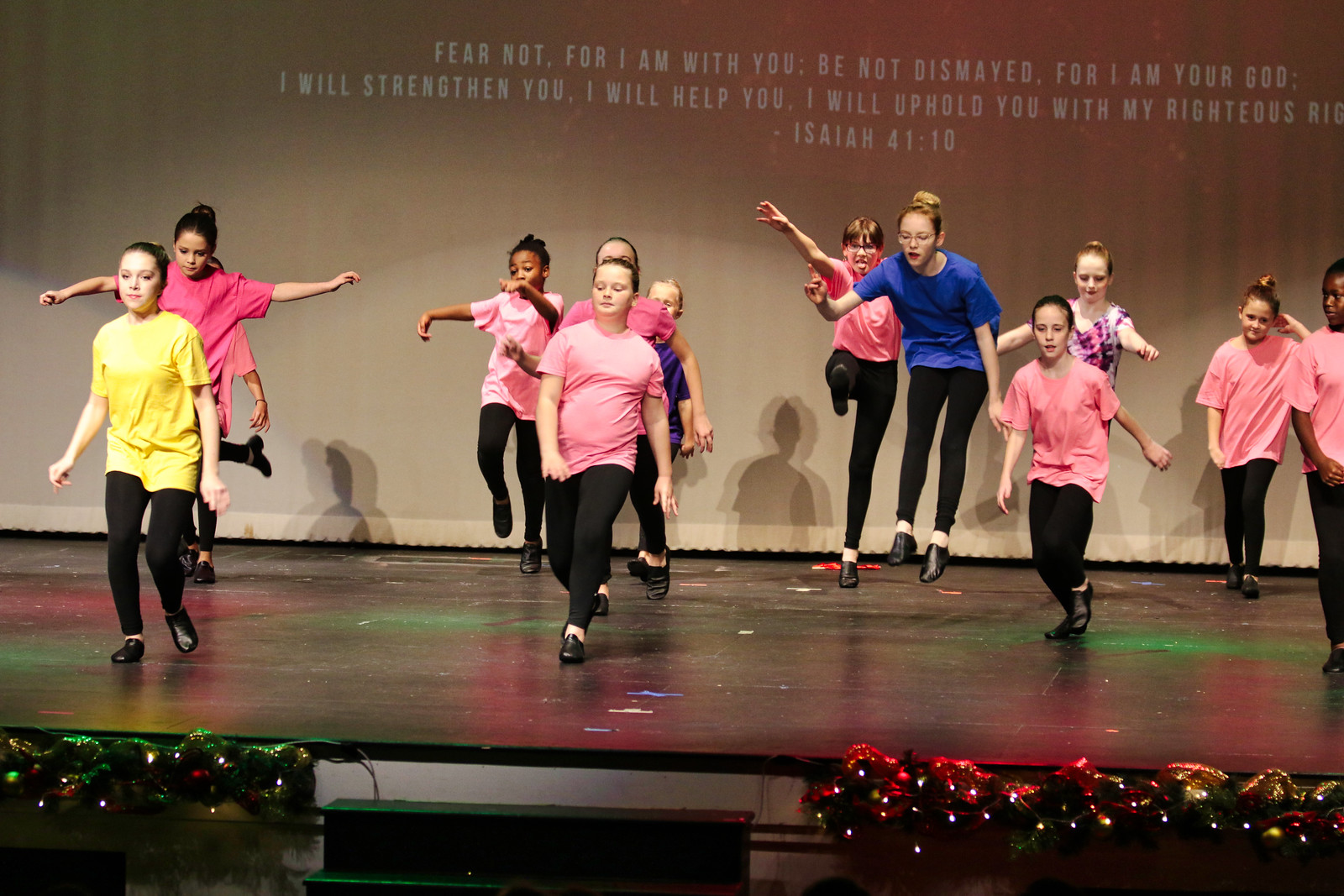The photograph captures a lively scene of teenage girls, likely aged 7 to 10, dancing on a brown stage adorned with Christmas lighting and festive wreaths, indicative of a holiday performance at a large church in the United States. The group of young girls, all wearing black tights and black shoes, is dressed in vibrant t-shirts, predominantly pink, with some donning yellow, blue, and a colorful tie-dye shirt. The backdrop of the stage features a prominent curtain or projector screen displaying a biblical quote in white text: "Fear not, for I am with you. Be not dismayed, for I am your God. I will strengthen you. I will help you. I will uphold you with my righteous right hand. Isaiah 41:10." The girls, arrayed in formation, seem to be enthusiastically performing individual dance moves, adding to the unchoreographed yet spirited atmosphere of the event.